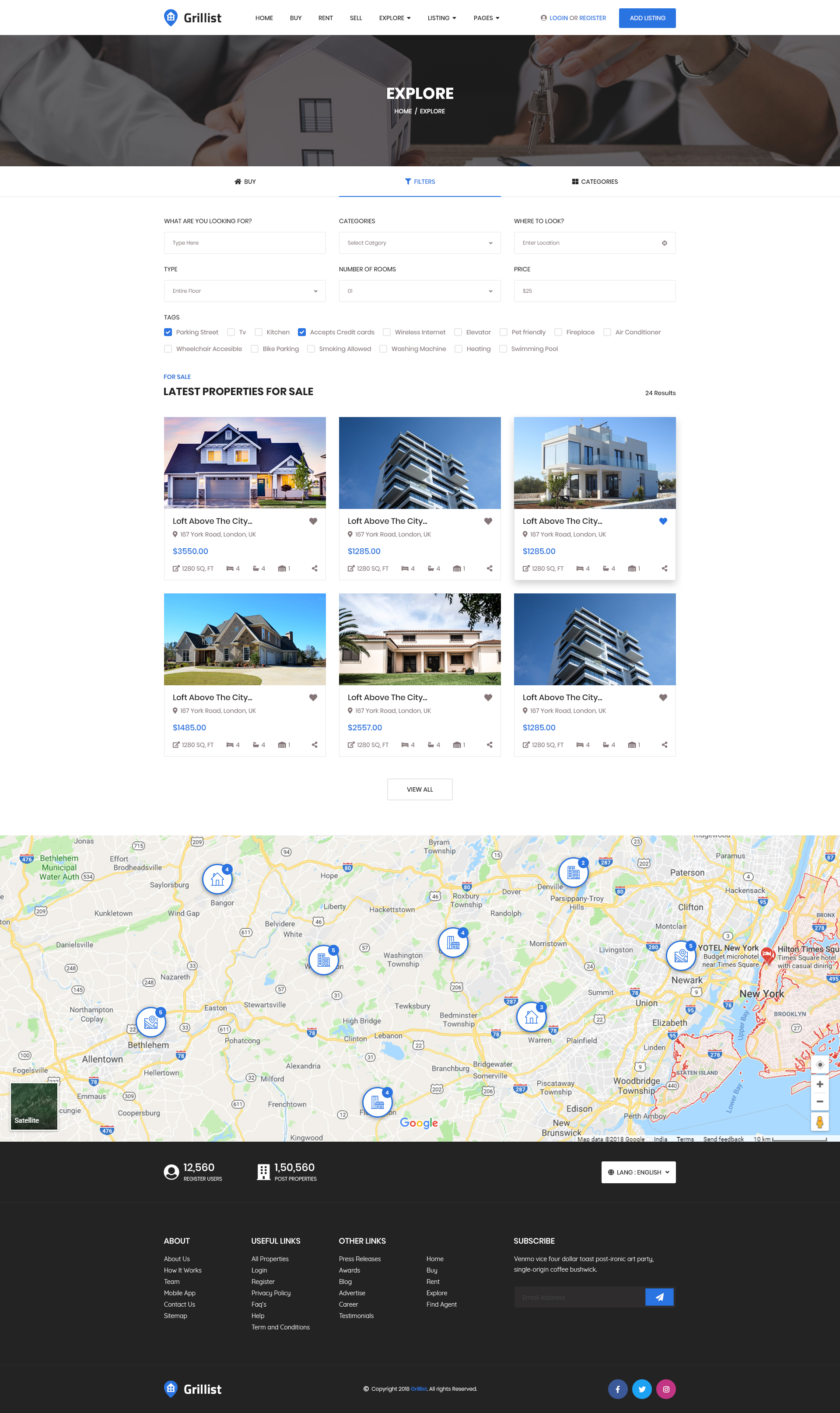Here is a detailed and cleaned-up descriptive caption for the image:

---

A vertically elongated image showcases a complete overview of a website, capturing its full length from top to bottom. The resolution of the text is too low to be readable, but the layout and main elements are discernible. 

At the top of the website is a blue logo accompanied by black text, likely the company name. Below the logo is a navigation menu featuring seven items, and a blue button is situated in the upper right corner.

A banner occupies approximately 10% of the total height beneath the navigation menu. This banner features a faded image of hands constructing a small model house on a wooden surface, with the house centered in the frame. The overlaying text on the banner reads "Explore" in white, with two additional unreadable words beneath it.

Following the banner, the webpage is divided into three columns against a white background. Each column has a heading, with the middle column's header highlighted in blue. These columns contain several lines of text, spanning about 20% of the image's height.

Further down, the section labeled "Latest Properties for Sale" is prominent. This section displays six images of different properties, each accompanied by brief descriptions underneath.

---

This caption provides a clear and detailed explanation of the visual content, making it easier for readers to understand the structure and elements of the webpage depicted in the image.